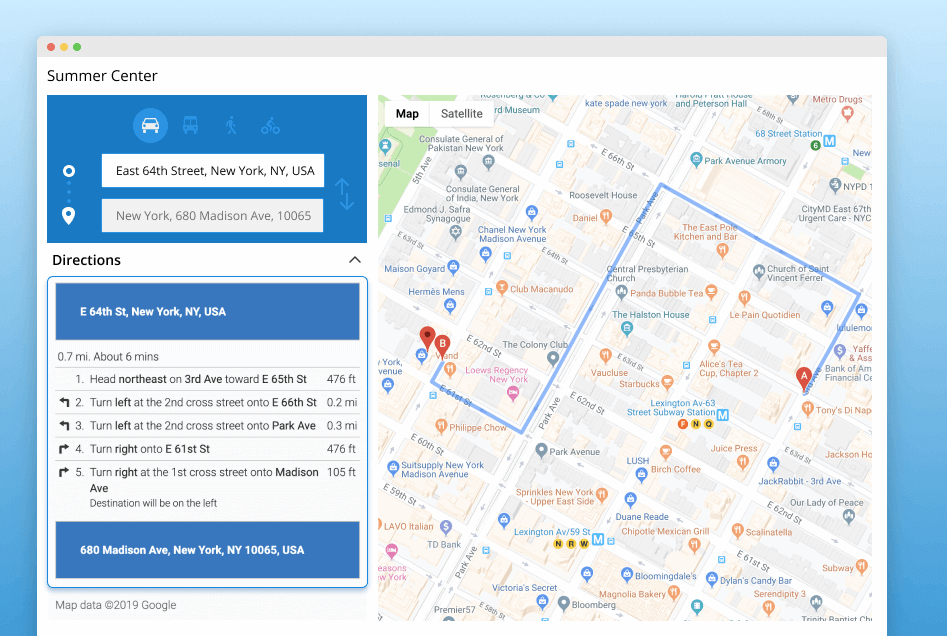The given image is a screenshot of a webpage displaying a detailed map. The map dominates the central section of the page and is set against a pale blue background. The map itself is primarily white, with an overlay of streets and paths. 

To the left of the map, there is a conspicuous blue and white frame that provides navigational instructions. At the top of this frame, the words "Summer Center" are written in bold black text. Above this title, three small circles are arranged horizontally, each in a distinct color - blue, red, yellow, and green. Beneath "Summer Center," there is a white rectangular background featuring the address: "East 64th Street, New York, New York, USA." Following the address, there are specific written directions in black text.

On the right side of the image, the map shows intricate details of intersecting streets, emphasizing an 'S'-shaped blue line. This line illustrates the route from the starting point, labeled 'B,' to the destination, pointed out as 'A'.